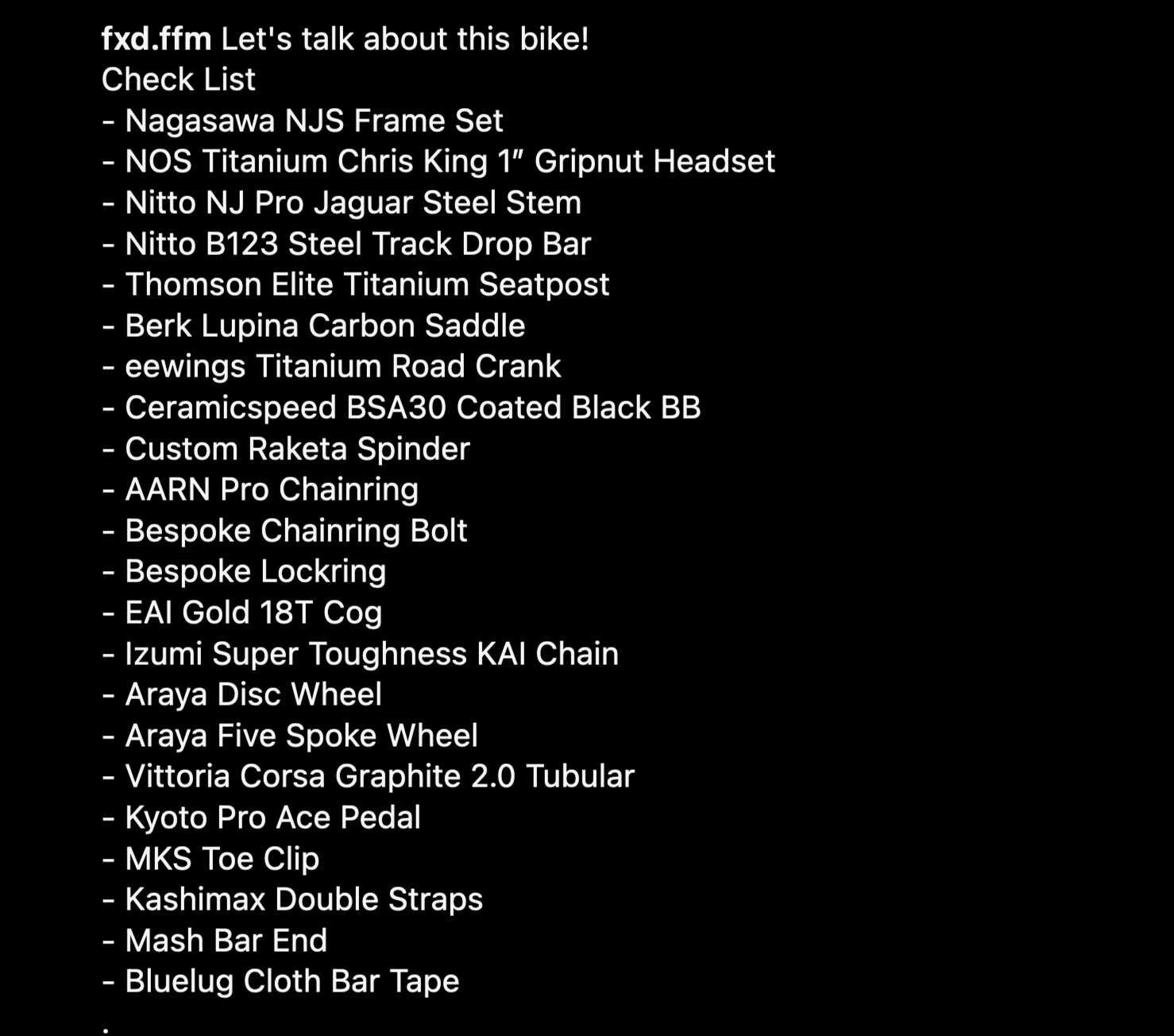The image features a minimalist design with several lines of small white text organized in a column against a solid black background. At the top, it begins with "fxd.ffmlet" followed by an emphatic "Let's talk about this bike!" Next, under the heading "Checklist," a bulleted list details various high-end components of the bicycle, including a Nagasawa NJS frameset, a NOS Titanium Chris King 1-inch grip nut headset, a Nitto NJ Pro Jaguar steel stem, a Nitto B123 steel track drop bar, a Thompson Elite titanium seat post, and a Burke Lupina carbon saddle. Additional notable features mentioned are a Ceramic Speed BSA 30 coated black bottom bracket, an Owings Titanium road crank, a custom Rikita spender, a bespoke chain ring bolt, and bespoke lock ring. The overall layout and font choice reflect a clean, graphic design typographic style.